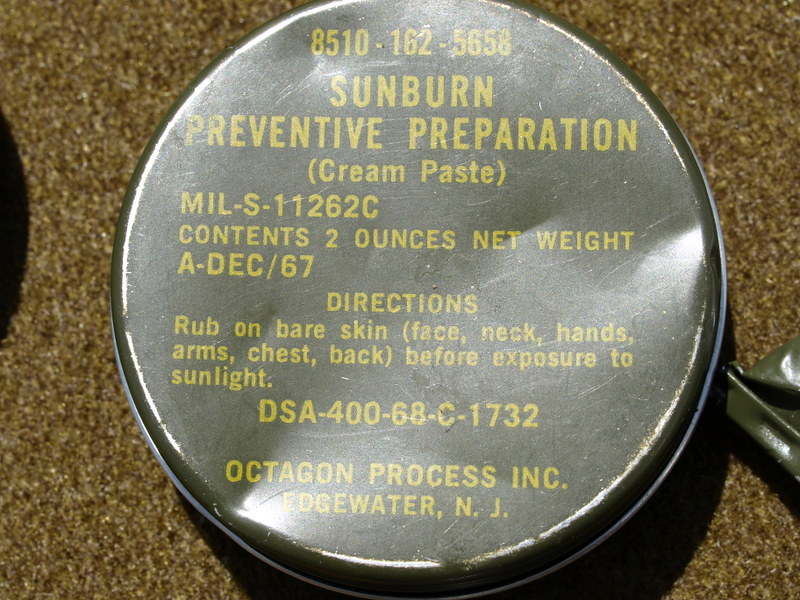The photograph depicts an old, weathered military green tin can with distinctive dents, positioned centrally on a brown carpet, set indoors. The tin is adorned with yellow text on its cover, including the numbers "8510-162-5658" followed by "Sunburn Preventative Preparation" and "MIL-S-11262C." The container has a net weight of 2 ounces and the date "A-DEC-67." Detailed usage instructions specify to "rub on bare skin (face, neck, hands, arms, chest, back) before exposure to sunlight." The bottom text reads "Octagon Process Incorporated, Edgewater, New Jersey," with the code "DSA-400-68-C-1732." This tin, likely a military-issued sunscreen, illustrates its age and historical usage.